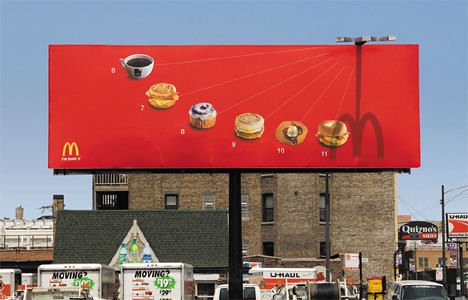In this real-life cityscape, the focus is a prominent McDonald's advertisement displayed high above the urban scene. The billboard features a red background showcasing six different food options, each labeled with a number starting from six. At number six, a coffee cup is depicted; number seven displays a sandwich; number eight appears to be a sweet dessert; number nine is another sandwich; number ten shows a pancake with syrup and butter; and number eleven features what seems to be a burger or another type of sandwich. Intriguingly, a metal fixture affixed to the top of the sign casts a shadow in the shape of the iconic McDonald's "M" logo. 

Below this striking advertisement, the city unfolds with a variety of structures and vehicles. A large, four-story brown building looms in the background, adjacent to another building characterized by its distinctive black roof. In the foreground, only the tops of several U-Haul vehicles are visible, some parked facing away to reveal their backs with white text indicating rental prices on a green background. Others are positioned sideways. To the right of the McDonald's sign, additional business signage is visible, including those for Quiznos and a U-Haul office. To the left, the upper portion of an industrial-looking building suggests a business area filled with shops and various establishments, contributing to the vibrant tapestry of this urban environment.